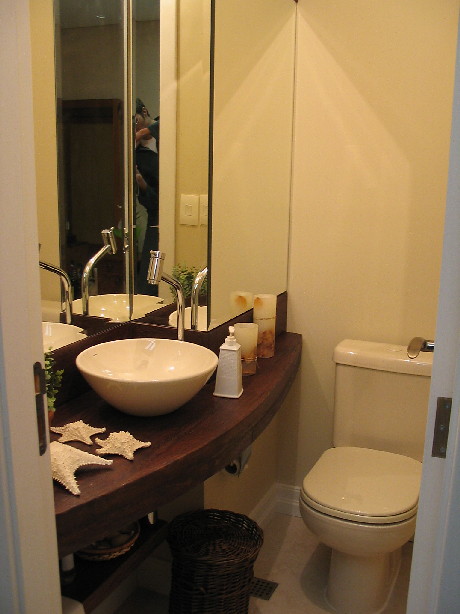In this warmly lit bathroom scene, the right side features a toilet with an oval-shaped seat in a down position. The toilet has a tank on the back with a rectangular rounded cap on top, and the whole unit exudes a yellowish tint. The background wall is a light brown, catching light reflections that converge near the top.

On the left side of the bathroom, a dark brown countertop is prominently displayed. Adorning the bottom left corner of this countertop are three starfish, with the largest at the bottom and two smaller ones positioned above it. Above these starfish sits a wide, white porcelain bowl that narrows towards the bottom. The bowl catches light reflections prominently in its center. 

Adjacent to the bowl is a white container holding a small white item, resembling a lit candle. Above the container are two candles, featuring cream-colored tops and brown floral designs at their bases. Farther to the left and slightly behind, a mirror reflects part of the room. The mirror is bordered by a black line, indicating it can slide apart, and it also has a gray line. Reflected in the mirror is a silver faucet, which is also visible directly behind the white bowl. Below this setup, there is a black trash can lined with a black bag.